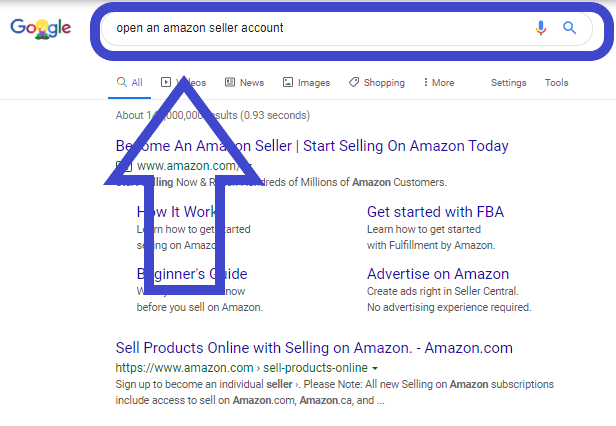The image depicts a Google search results page with a white background. In the upper left corner, the recognizable Google logo is prominently displayed. Centered below the logo is the search bar, which contains the query: "Open an Amazon Seller Account." Just underneath the search bar, the default filter is set to "All," but other options like "Videos," "News," "Images," "Shopping," and "More" are also available. To the right, there are quick access links labeled "Settings" and "Tools."

In the main body of the page, the search results begin, stating there are approximately one million results, which were generated in 0.93 seconds. The first search result features a blue title: "Become an Amazon Seller, Start Selling on Amazon Today," followed by a green URL link to Amazon.com. Below this link are four categorized quick links facilitating direct navigation: "How It Works," "Beginner Guide," "Get Started with FBA," and "Advertise on Amazon." Each of these sections includes a brief description, providing a more detailed pathway to specific parts of the Amazon seller information page.